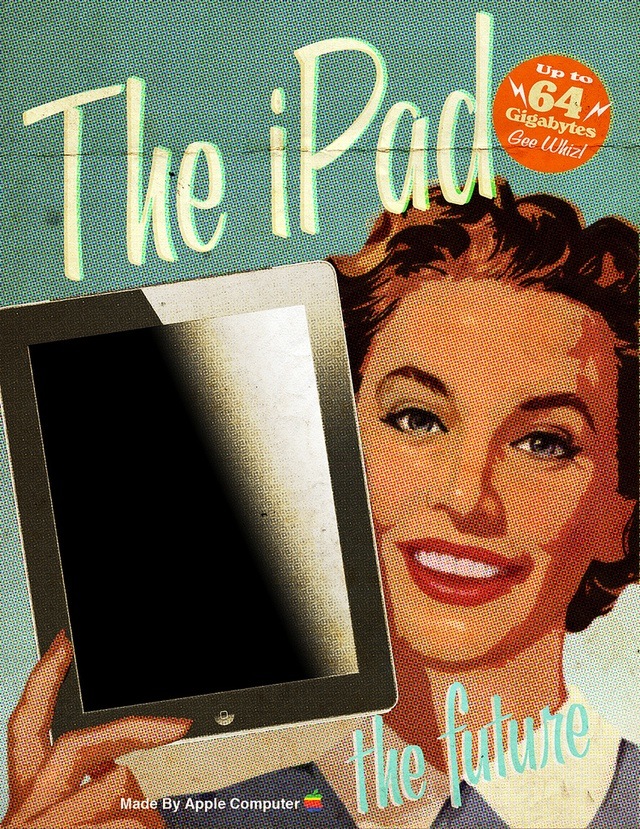This image is a modern advertisement for the iPad, designed with a retro flair reminiscent of the 1950s. The entire picture is rendered with a dot matrix pattern and screen-print texture, enhancing its old-fashioned appearance. At the center stands a woman with short brown hair, a white collar, and a blue top, smiling as she holds the iPad up near her face. The ad features a playful, retro font, proclaiming phrases such as "Made by Apple Computer," "The Future," and "Up to 64 gigabytes, Gee Whiz!" Additionally, there are two tiny lightning bolts beside the storage claim, and the iPad screen has a grainy, gradated look to match the vintage aesthetic. The overall color palette consists of dusty, muted hues, completing the nostalgic design.